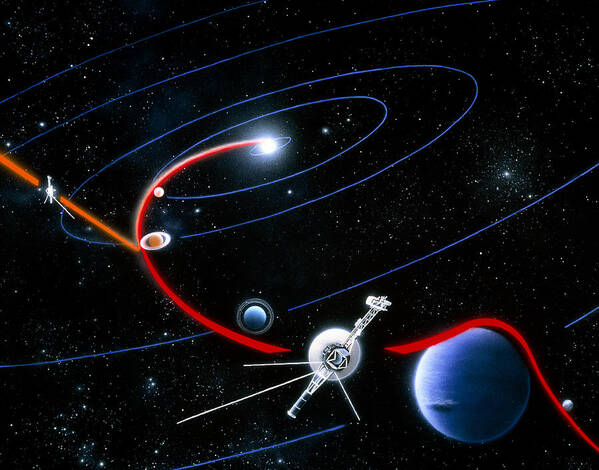This is an artistic drawing depicting a satellite's path through outer space. The image features a square-shaped composition with a predominantly black background, speckled with white dots representing distant stars and planets. At the center, a large white star, presumably the sun, emanates a red line extending outward. Positioned along this red line is a sizable satellite, designed with a white framework and an extensive white satellite dish, from which three lines extend downward. 

Additionally, an orange line diverges in a different direction from the red line's path. Surrounding the central star are several large blue circles, indicating planetary rotations, with each circle increasing in size the farther it is from the center. Notable elements include a large blue planet with an encircling red line, which symbolizes its orbit.

The drawing also features another space station or spacecraft detailed with a circular design located towards the middle, showcasing the complexity and intricacies of space exploration equipment. The image captures the dynamic and layered nature of outer space, blending scientific accuracy with artistic expression.